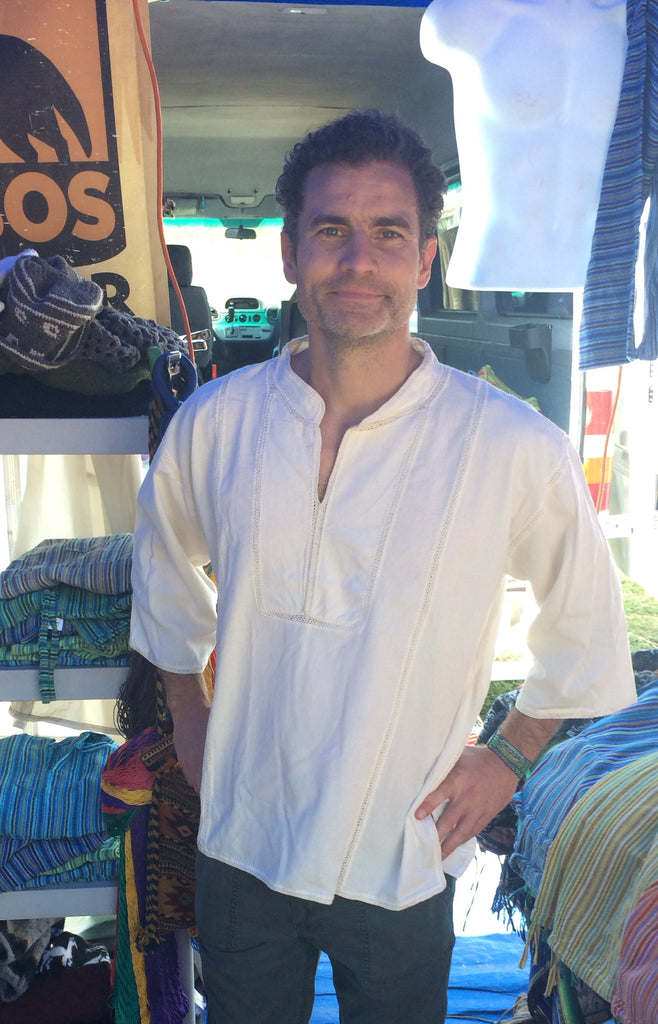The image showcases a man standing and looking directly at the camera. He has short, curly dark hair, thick brown eyebrows, and is clean-shaven with a slight smile. He is wearing a white half-sleeve shirt, reminiscent of a poet shirt, paired with gray pants. His hands rest by his thighs, one adorned with a green bracelet. The background reveals the interior of a vehicle, possibly a truck or a minivan, with an open door allowing light to stream in. Surrounding him on both sides are shelves filled with an array of colorful striped fabrics, including shades of blue, green, red, and various other colors, indicating that he is in a setting resembling an outdoor swap meet or market. To his left, there's a shelf stocked with clothing and other materials, while a table on his right holds more fabric pieces. The overall scene is illuminated by natural light coming through the vehicle’s front window.